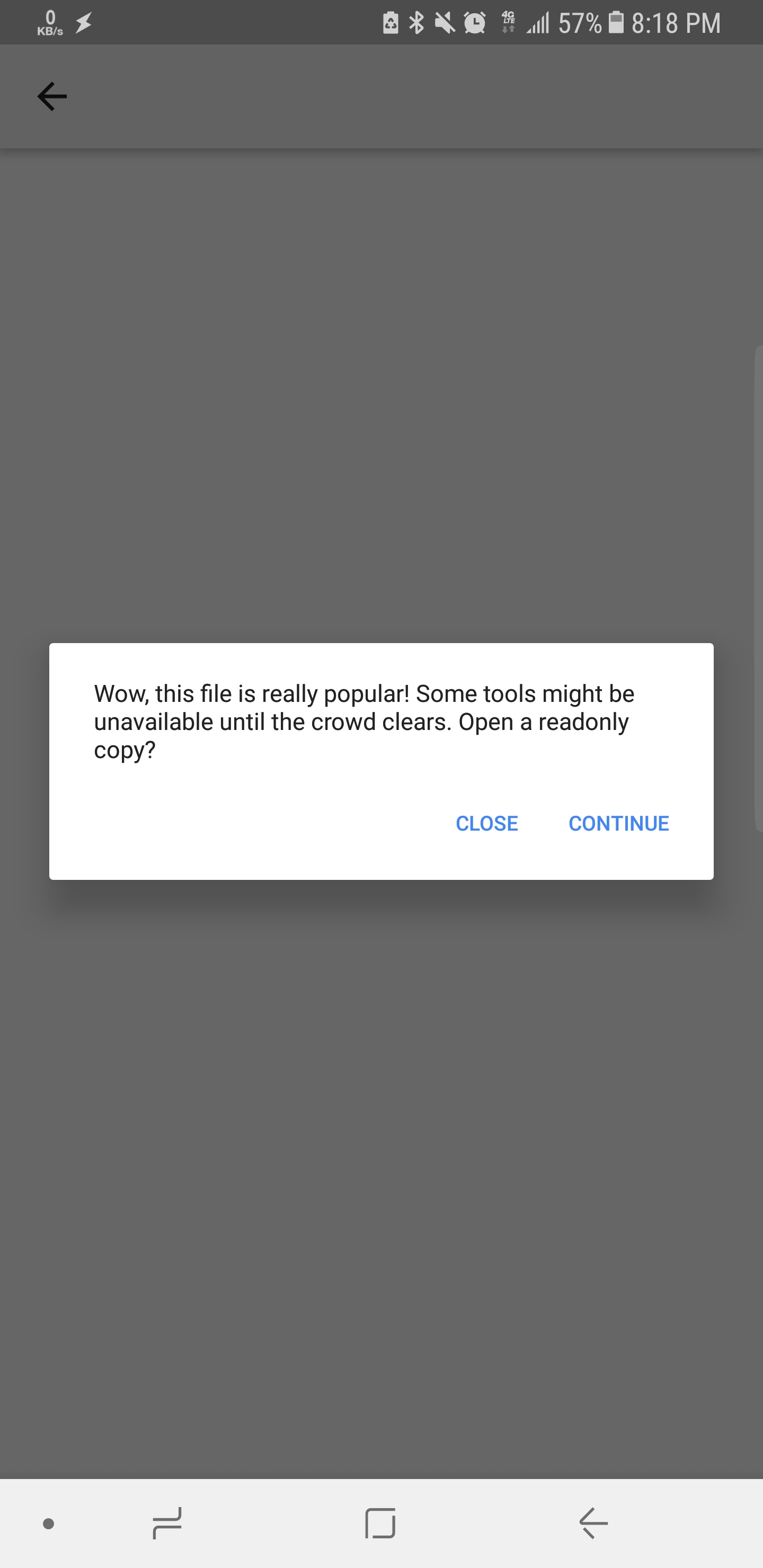Screenshot of an app message in progress displays various status icons at the top, starting from a signal strength icon, followed by a flash icon, a battery icon, a Bluetooth icon, an audio icon, a clock icon, a download/upload icon, network bars, a percentage indicator showing 57% battery life, and a timestamp indicating 8:18 PM. Below these icons, an arrow points to the right. The central part of the screenshot features a message within a white rectangular box that says, "Wow, this file is really popular. Some tools might be unavailable until the crowd clears. Open a read-only copy?" Below the message, there are two options: "Close" and "Continue."